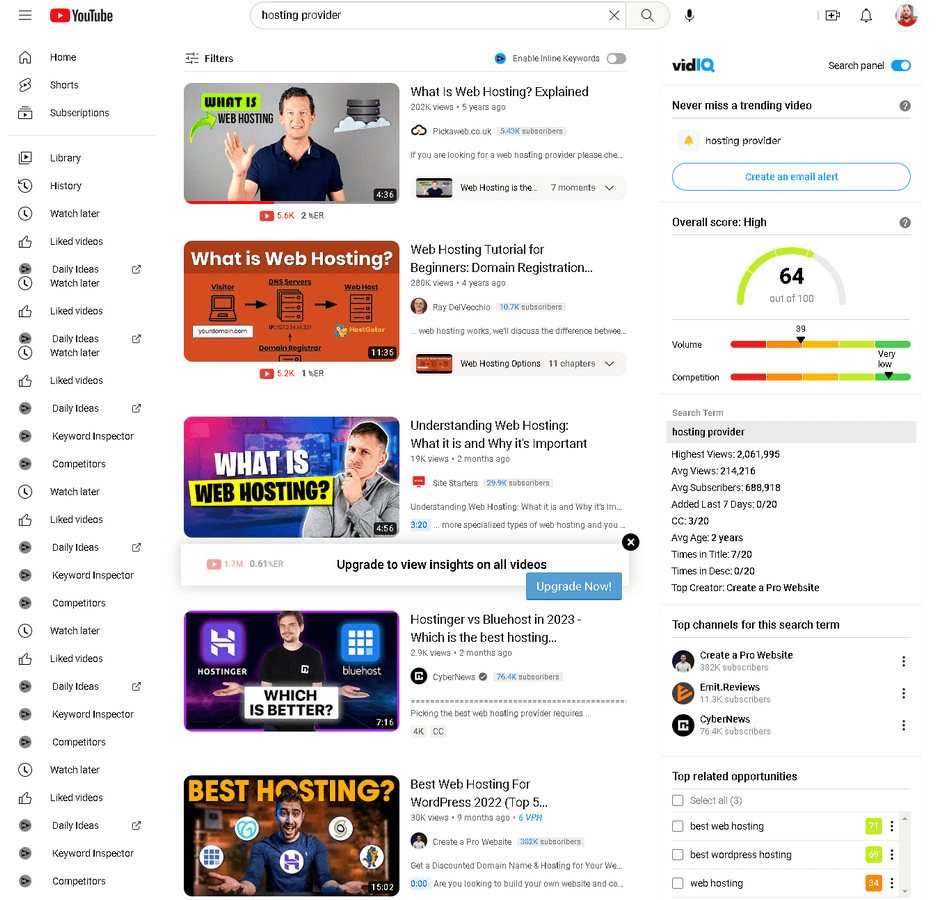**Detailed Caption:**

The image captures a screenshot of the YouTube website, prominently displayed under the heading "Websites." The top part of the page features a search bar with the phrase "hosting provider" entered. On the left sidebar, several navigation options are listed: Home, Shorts, Subscriptions, Library, History, Watch Later, Liked Videos, Daily Ideas, Watch Later, Keyword Inspector, and Competitors.

To the right of this sidebar, various video thumbnails are presented. The first video thumbnail features a man in a blue collared shirt with an orange background, indicating the title "What is Web Hosting." The background also includes graphical representations of a computer, DNS servers, and web hosts.

Below this, another thumbnail shows a man in a gray shirt with his finger on his chin, striking a contemplative pose. This video is titled "Which is better: Hostinger or Bluehost?" labeled with "Best Hosting" underneath.

The detailed layout and contents of the YouTube page reflect an emphasis on tutorials and comparative reviews related to web hosting.